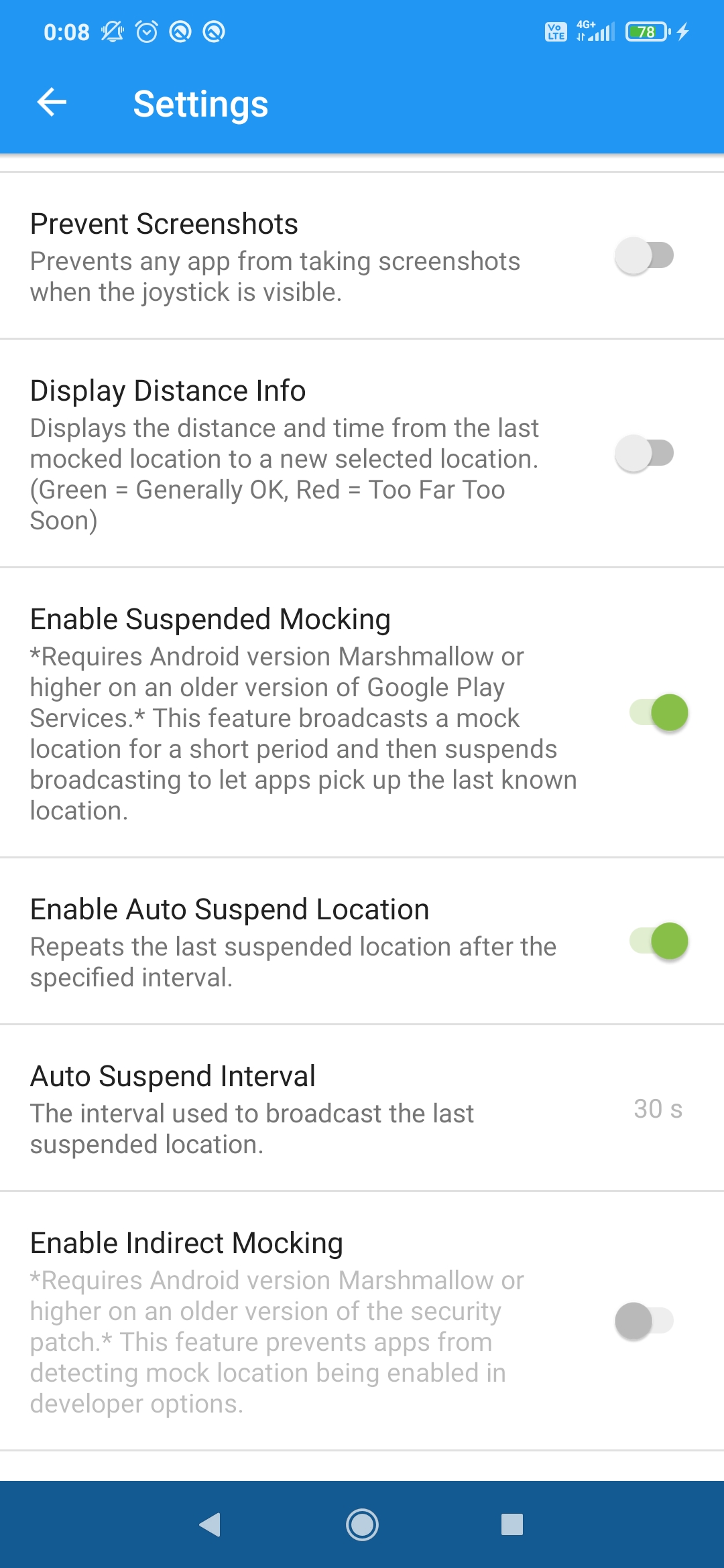In the provided image, which is a screenshot of a phone screen, various details and elements are distinctly visible. At the very top, within a blue bordered area, several status icons can be seen. On the far right, there is a battery icon displaying the number "78" in green text, indicating the battery percentage. Adjacent to it, a lightning icon signifies that the phone is charging. Moving leftward, the phone signal strength icon shows 4 out of 5 bars. Further left, within a white box, the text "LTE" indicates the type of mobile data connection. On the far left, the current time is displayed as "0:08."

Next to the time are several icons: a bell icon with a slash through it indicating notifications are silenced, an alarm clock icon, and two circular icons with similar designs. To the right of these icons, the word "Settings" is visible, with an arrow pointing left, suggesting a return to the previous settings page.

Below this top section, there are several categories listed in descending order: "Prevent screenshots," "Display distance info," "Enable suspended mocking," "Enable auto suspend location," "Auto suspend interval," and "Enable indirect mocking." Each of these represents different configurable settings.

At the very bottom of the image, within a dark blue border, the navigation buttons are shown: a back button, a home circle button, and a square button for recent apps. These buttons are colored in a grayish hue.